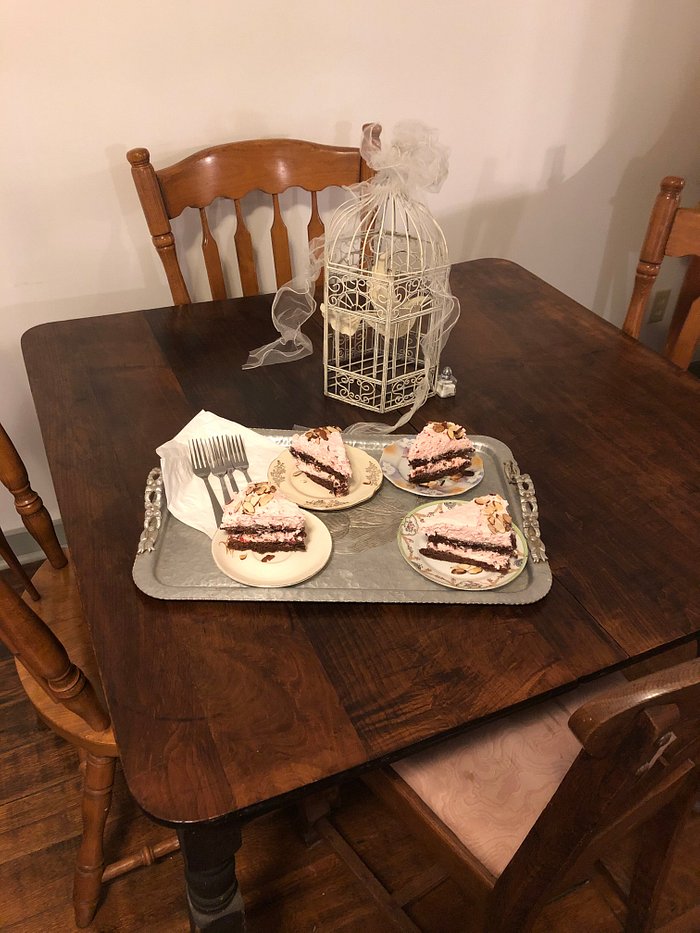The photo depicts an Americana-style dining room with rich, dark brown and black wooden floors. At the center is a square wooden dining table, sharing a similar dark brown and black hue, surrounded by four light brown wooden chairs. Each chair features wooden posts on the back, four sturdy legs, and support beams. Positioned in the bottom right corner is a distinct chair, characterized by a flat wooden back and a padded white cushion on the seat. The backdrop is a soft, off-white wall, enhancing the room's classic feel.

Prominently placed on the table is a decorative white metal birdcage adorned with intricate embroideries and a translucent white ribbon. Next to the birdcage sits a small see-through salt shaker containing white granules. In front of the birdcage lies a rectangular silver metal platter holding a folded white napkin and four silver forks. Arranged on the platter are four plates, each containing a slice of a multi-layered cake/pie. The dessert features alternating layers of tan crust and dark blue blueberry filling, typical of a blueberry pie, though some descriptions hint at chocolate and pink frosting variations with nut slices on top. The plates themselves showcase diverse patterns, including white with blue embroidery designs, adding a touch of elegance to the rustic setting.